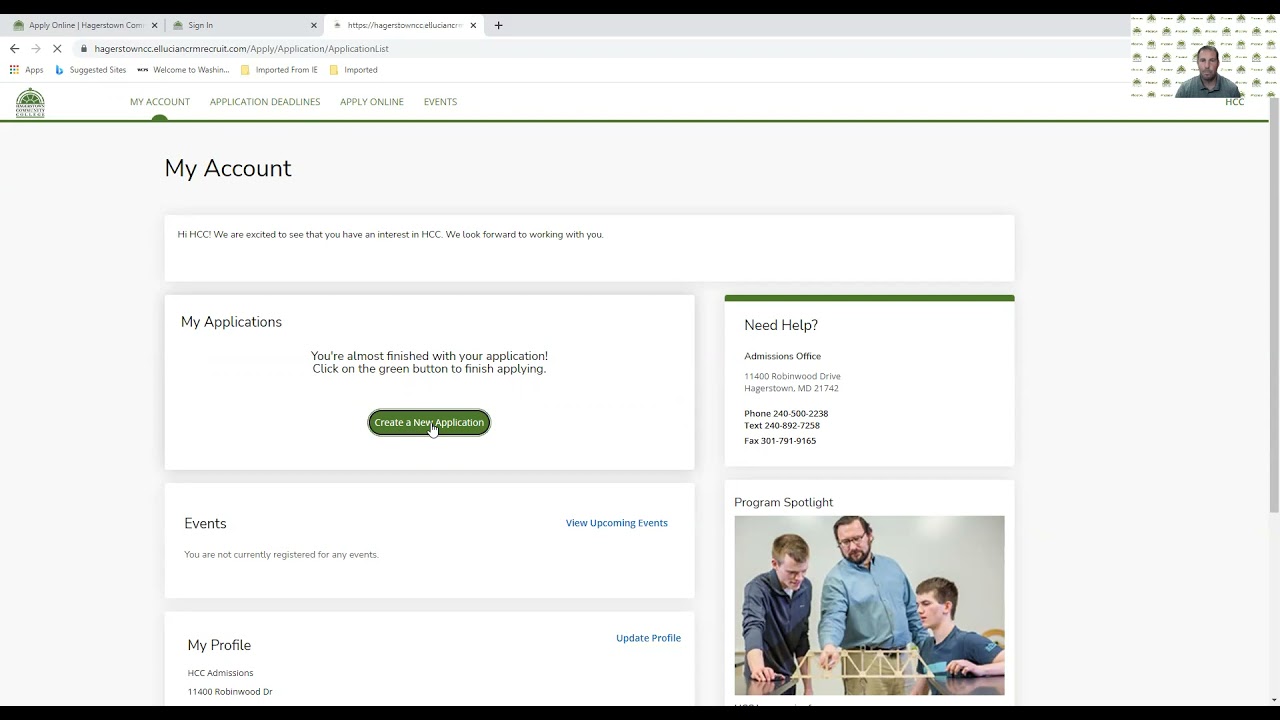The image showcases a webpage from the Hagerstown Community College recruitment portal, specifically the application dashboard. The URL in the taskbar reads "hagerstowncc.illusioncrmrecruit.com/apply/application/application-list," indicating that this is a site for prospective applicants. At the top of the page, navigation tabs are visible, including "My Account," "Application Deadlines," "Apply Online," and "Events."

Just below the navigation tabs, there is a welcoming message: "My Account: Hi HCC, we are excited to see that you have an interest in HCC. We look forward to working with you." Below this, a section titled "My Applications" prompts the user to complete their application with a notice that says, "You're almost finished with your application. Click on the green button to finish applying." A prominent green button labeled "Create New Application" invites the user to proceed.

To the left, there is a box titled "Events," and at the bottom, there's another box labeled "My Profile." On the right side of the page, there's a "Need Help" box that provides contact information for user assistance. The layout is organized to facilitate easy navigation for users to manage their application process efficiently.